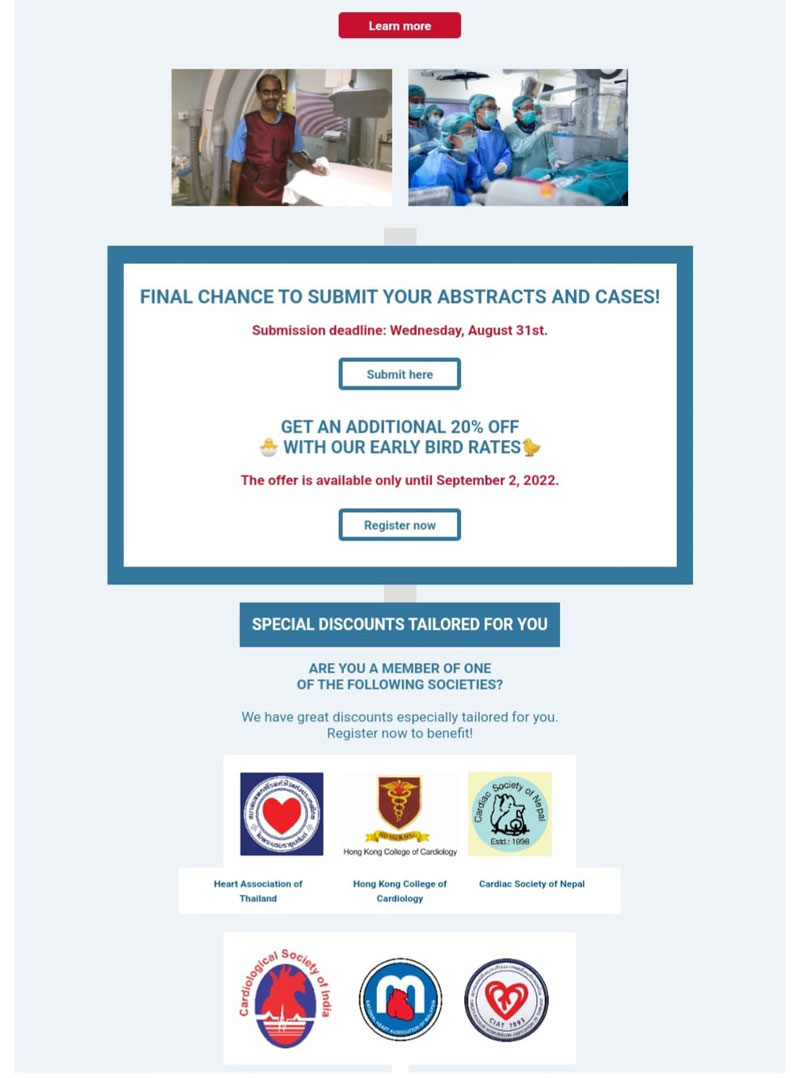This image, captured from a web page, features two medical-themed photographs at the top and a promotional section below them. 

On the left, a small inset photo displays a radiology technician, possibly of Black or Indian descent, dressed in a blue shirt and a red protective lead suit. He is positioned beside a white table, likely part of a CT (CAT) scan machine, suggesting a clinical setting.

To the right, another image shows an operating room with five individuals wearing masks. They are interacting with a ceiling-mounted device, which appears to be an x-ray machine, positioned over an area where a patient might lie.

Below these images, a prominent box with a blue outline includes various text elements. In blue letters, it reads, "Final chance to submit your abstracts and cases," followed by "Submission deadline: Wednesday, August 31st" in red. A "Submit Here" button is also present. Beneath this, there is a note about receiving an additional 20% discount with early bird rates. In red, it warns that this offer is available only until September 2nd, 2022. A "Register Now" button is situated below this information.

Outside this larger box, a separate button labeled "Special Discounts Tailored for You" appears. Below this, it asks if the viewer is a member of one of the displayed societies, which are represented by six logos.

The entire layout is aimed at encouraging prompt submission of medical abstracts and cases, while also offering incentives for early registration.